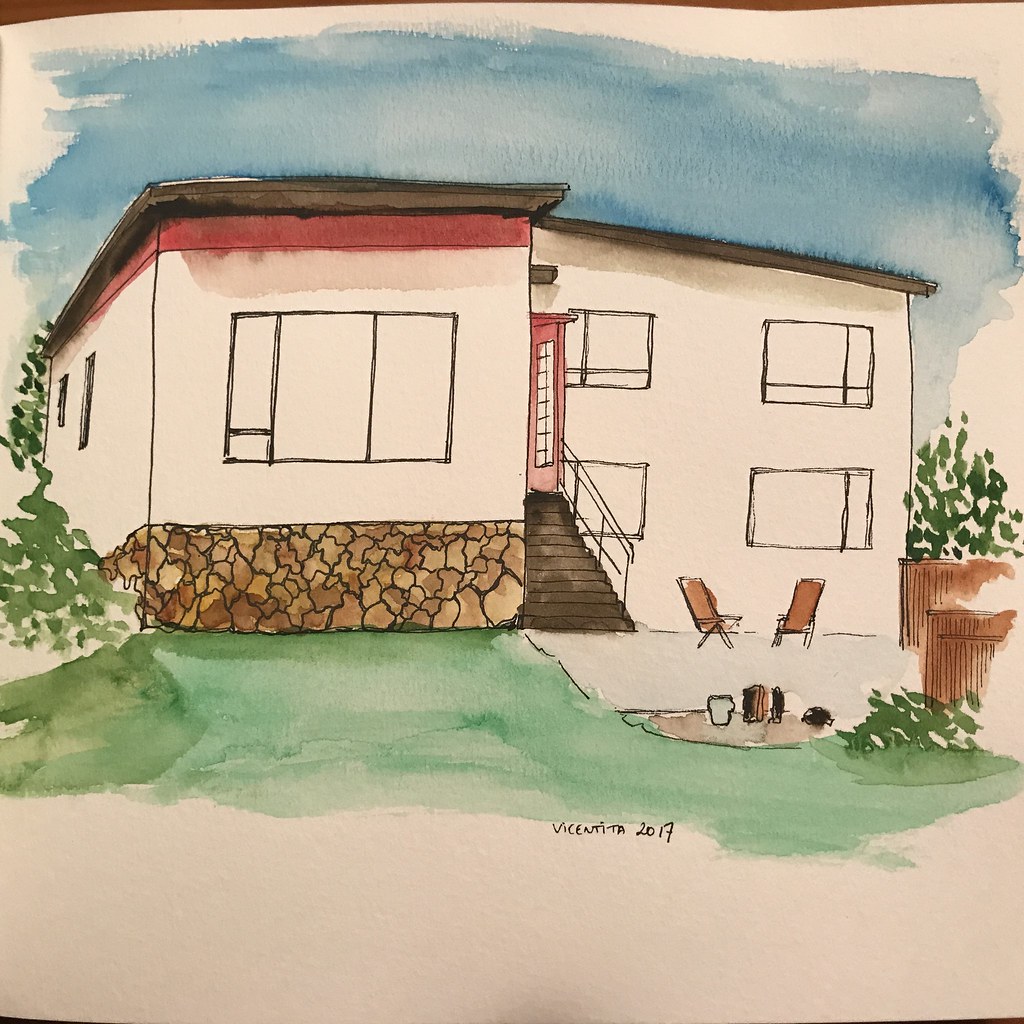This detailed watercolor painting captures a contemporary house with a mix of modern and traditional elements. The left side of the house is a single story, featuring a prominent front window framed by brown stone at the base, with a bold red panel above it. The roof is brown, and two small windows are positioned on the left side. Adjacent to this section, on the right, a two-story structure showcases a red door centrally located with brown stairs leading up to it, supported by a black railing. This part of the house features four distinct windows and a matching brown roof. The backdrop is a clear blue sky, enhancing the overall aesthetic.

Flanking the house are vibrant green shrubs, and a brown fence demarcates the boundaries. At the base of the stairs, two brown chairs face each other, inviting a sense of hospitality. The yard is divided into a sandy area with a few scattered items and a lush green lawn. The artist, Vicentita, signed the piece in 2017. Below the grass, there's a large section left blank, its off-white hue creating a stark contrast with the rest of the vibrant scene.